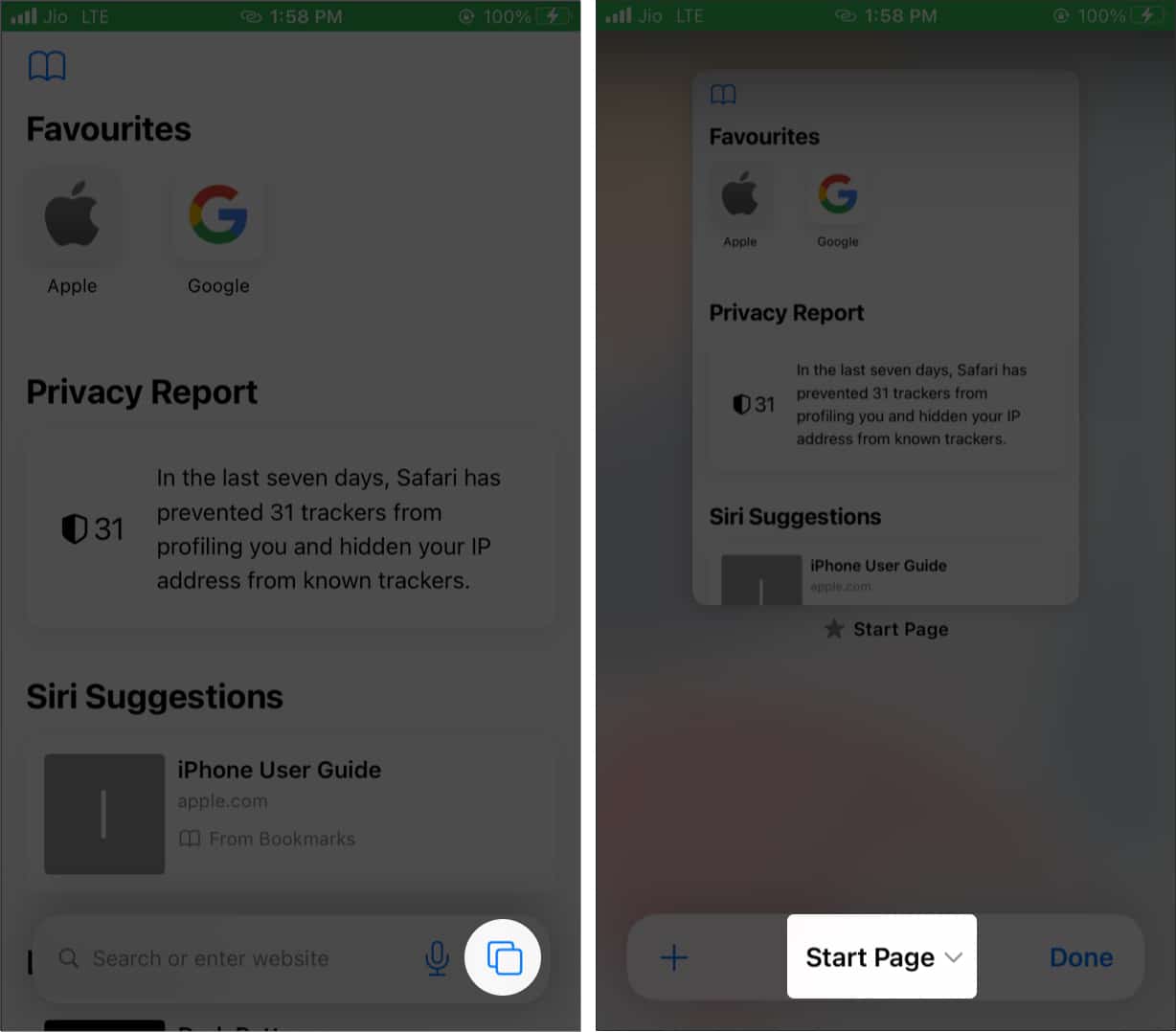This image features two screenshots from an Apple iPhone, showcasing a tutorial on how to use certain features in Safari. 

In the first screenshot, the screen displays a Safari browser with a white background. The page is slightly grayed out, with a small white circle at the bottom highlighting the "Copy Link" icon. The user interface lists Apple and Google as favorites, alongside a privacy report stating, "In the last seven days, Safari has prevented 31 trackers from profiling you and hidden your IP address from unknown trackers." Additional elements include Siri suggestions and an iPhone user guide, with a search bar labeled "Search or enter website name" located at the top.

The second screenshot retains the grayed-out background effect, but this time it highlights the "Start Page" button at the bottom of the screen. The screen also shows a shrunken version of the Safari page, similar to the animation when closing a tab on an iPhone. Adjacent to the "Start Page" indicator is the word "Done," and a small plus icon is situated on the opposite side.

Overall, these screenshots collectively guide the user through a specific action or feature within the Safari browser, confirming that the images are part of a tutorial.